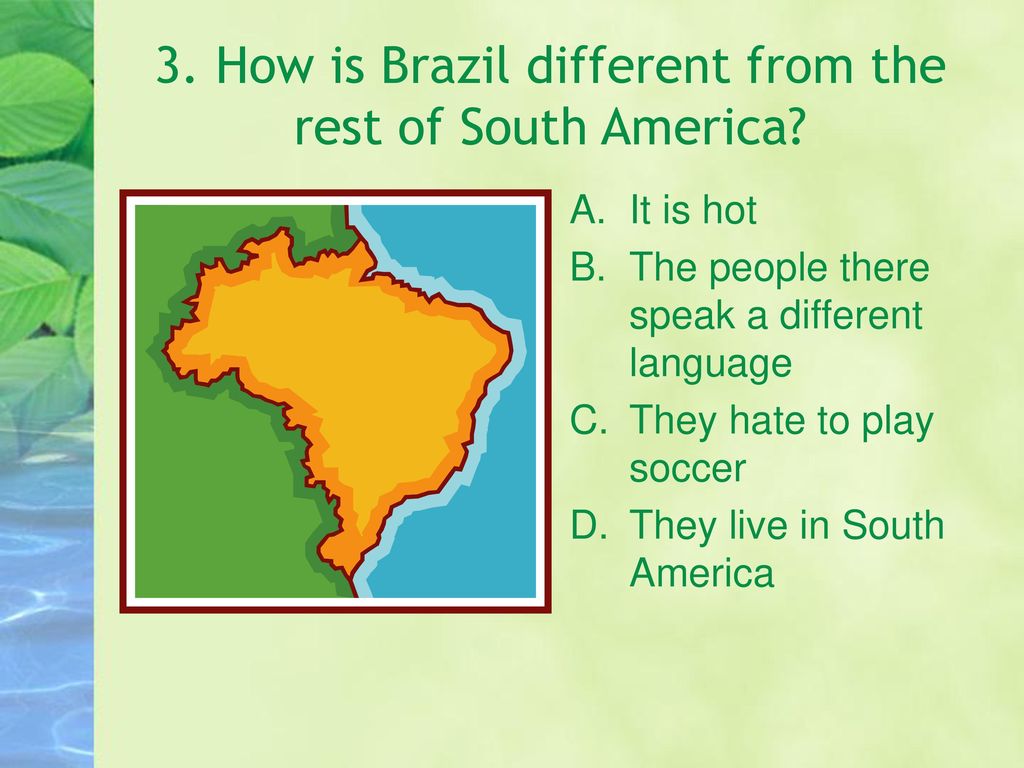The image features a predominantly green-themed page, with the most prominent element being a bold green headline at the top. The headline reads: "Three Dots: How is Brazil Different from the Rest of South America?" Below the headline, a list of multiple-choice options labeled A to D is presented in green text. The options are:

A. It is hot
B. The people there speak a different language
C. They hate to play soccer
D. They live in South America

To the right of the text, a graphic design illustration depicts Brazil. The illustration showcases Brazil as a yellow-orange colored country with a red border. Surrounding Brazil, the graphic features a green landmass to the left and a blue area to the right, symbolizing adjacent water bodies. Additionally, on the left side of the image, there is a vertical strip adorned with green leaves at the top and a water scene with reflections at the bottom, adding a naturalistic touch to the composition. The entire graphic is framed with a red box-border and a white border, accentuating the visual details.